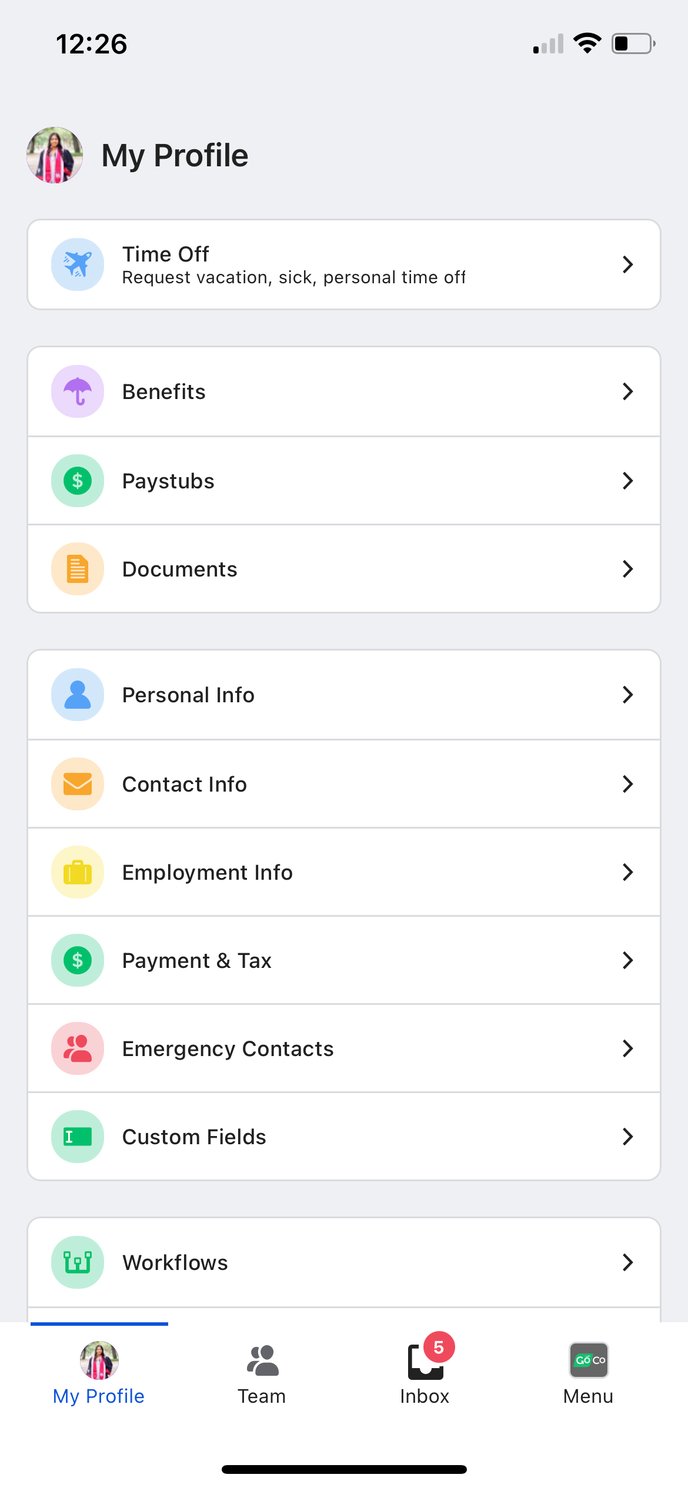A screenshot taken from a cell phone at 12:26 PM shows a user interface with a low wireless signal and a half-charged battery. At the top left, there is a small circular profile picture of a woman wearing what appears to be a purple and pink jacket or sweater. Next to the profile picture, the label "My Profile" is displayed.

Below, there's a box featuring a plane icon labeled "Time Off," which includes options for requesting vacation, sick leave, and personal time off, accompanied by a dropdown arrow to expand the menu. 

The next section comprises three menu items:
1. A purple icon with an umbrella labeled "Benefits," complete with a dropdown arrow.
2. A green circle with a dollar sign labeled "Pay Stubs," also featuring a dropdown arrow.
3. A yellow circle with a document icon labeled "Documents," again with a dropdown arrow.

Following this, another section contains six items:
1. A circle with a generic profile silhouette labeled "Personal Info" and a dropdown arrow.
2. An orange-yellow circle with an envelope icon labeled "Contact Info" and a dropdown arrow.
3. A brighter yellow circle showing what appears to be a suitcase, labeled "Employment Info," with a dropdown arrow.
4. A green circle with a dollar sign, similar to Pay Stubs, labeled "Payments and Tax," including a dropdown arrow.
5. A light red circle with two people icons labeled "Emergency Contacts," and a dropdown arrow.
6. A green circle with an eye icon labeled "Custom Fields," accompanied by a dropdown arrow.

The section further down begins with "Workflows," symbolized by a green circle featuring an icon resembling an elongated letter 'E' or a person with arms raised, with a dropdown arrow next to it.

The "My Profile" section is selected, showcasing the same profile picture as at the top. Next to this, there's an icon with two people labeled "Team," followed by an icon of a square with a '5' in a red circle indicating notifications, labeled "Inbox." At the far right, there is a black icon with green letters, difficult to decipher at this size, labeled "Menu."